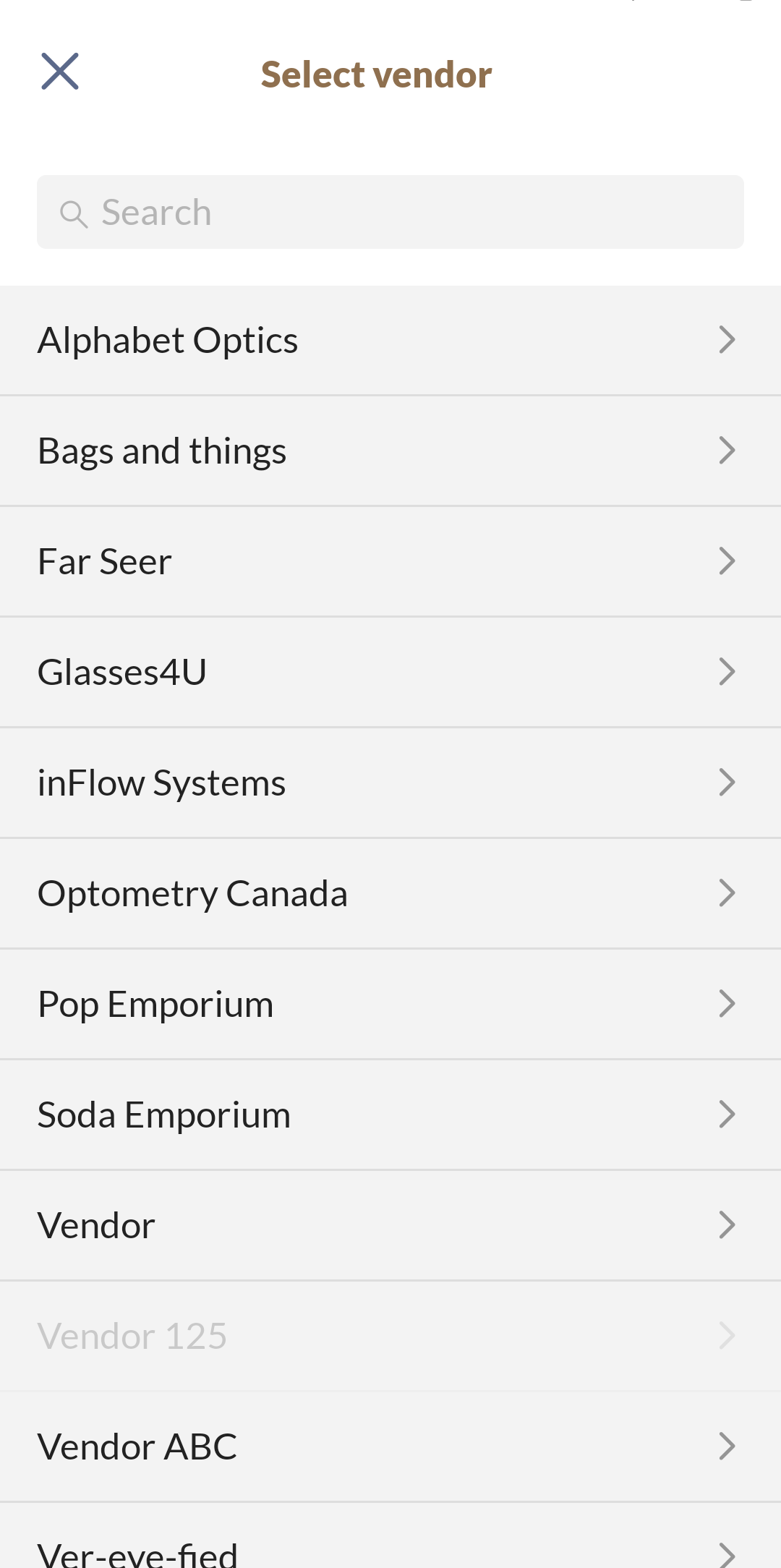The image displays a digital interface, likely part of an online platform for selecting vendors. At the top of the screen is a search bar labeled "Select Vendor" with a clickable icon next to it, possibly indicating a filter or menu option. Directly below the search bar is a comprehensive list of vendors arranged in a vertical column. Each vendor name is accompanied by an arrow icon, suggesting that clicking it will reveal additional options or details.

The list includes:
1. Alphabet Optics
2. Bags and Things for Our Seer
3. Glasses For You
4. Inflow Systems
5. Optometry Canada
6. Pop Emporium
7. Soda Emporium
8. Vendor 125
9. Vendor ABC
10. Ver I-5

The described interface is streamlined for easy navigation and clearly aimed at users seeking vendor-related information, potentially focusing on eyewear and beverage options.